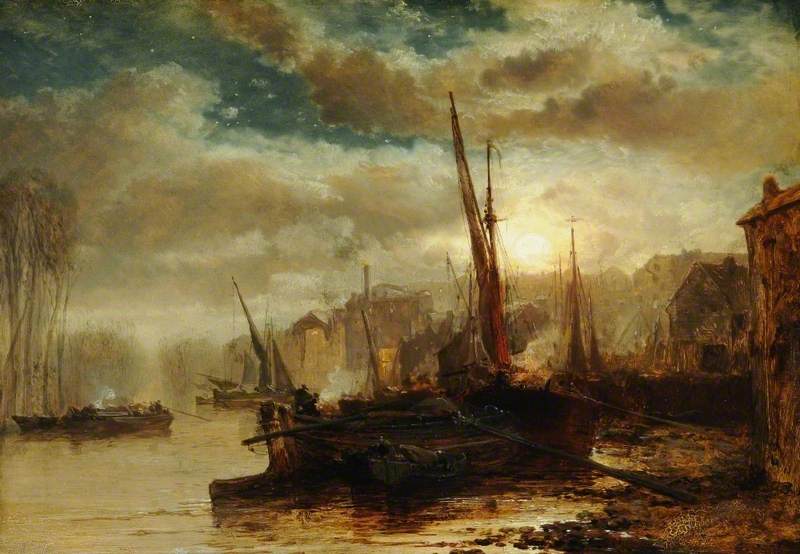This dramatic painting, evocative of the Dutch Renaissance style with an impressionistic twist, captures a war-torn town along a canal at dusk. The central focus is a barge or boat with a partially unfurled red sail on its staff, sitting on dark, reflective waters at the center of the image. To the left, smaller boats—some upended and others floating—populate the river near the desolation. In the distance, larger boats seem to be moving away from the devastated town, where several buildings on the right side stand dilapidated, charred, and engulfed in flames, contributing to an intense, almost war-zone atmosphere. The sky above is a moody, cloud-covered expanse with hints of dark blue, partially obscuring the setting sun and casting a haunting glow over the scene. The ominous clouds and the faint twinkle of stars enhance the painting's dramatic tension, merging the somber elements into a cohesive depiction of ruin and resilience.